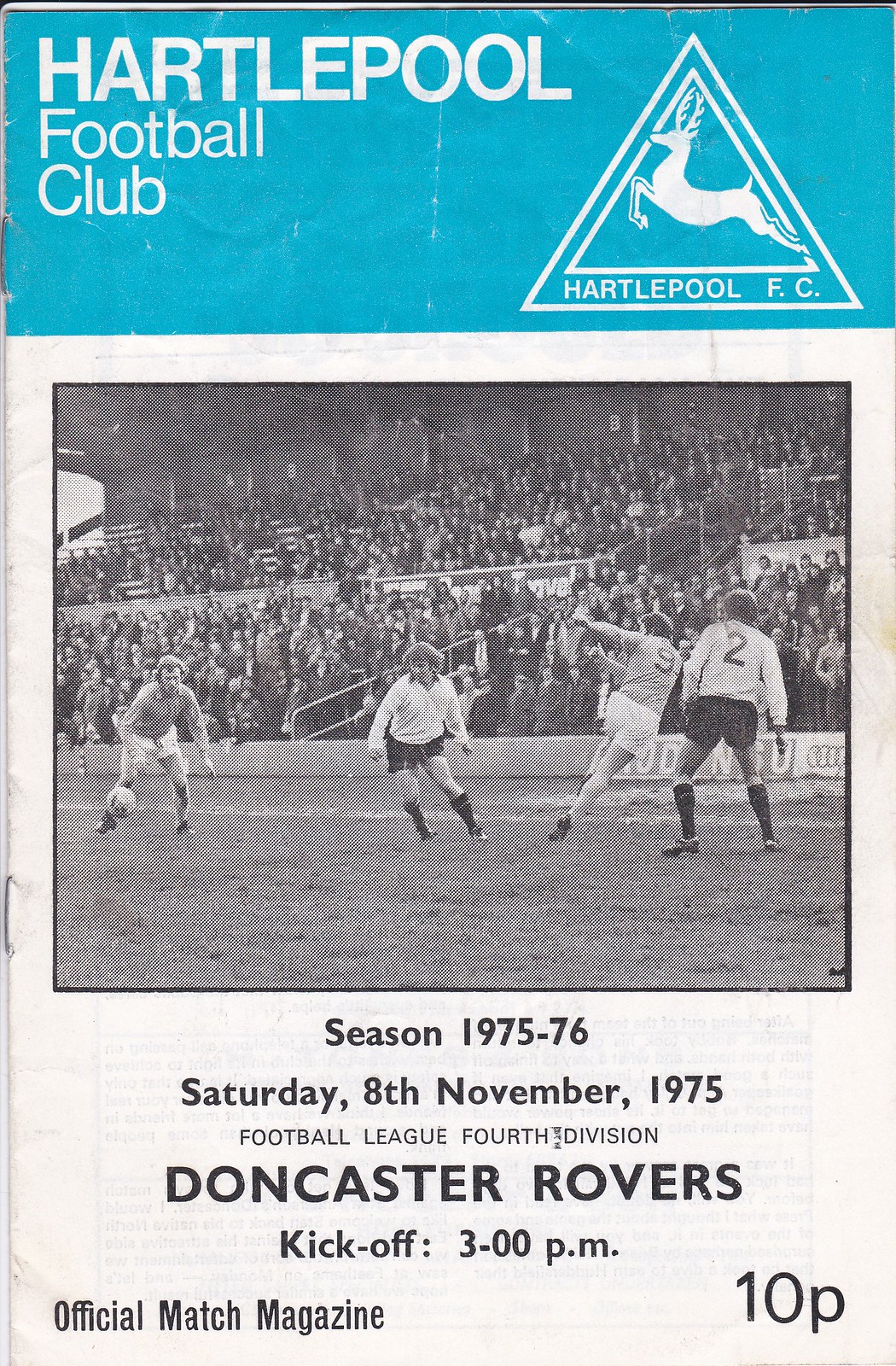This image features the cover of an official match program for a soccer match between Hartlepool Football Club and Doncaster Rovers that took place on November 8, 1975. The top 20% of the cover is dominated by a light blue banner with white block lettering that reads "Hartlepool Football Club." To the right of this text, set against the same light blue background, is the club's logo, a white silhouette of a jumping stag with many antlers, enclosed within two nested triangles. Below this, a faded black and white photograph depicts four soccer players in action on the field, with spectators visible in the packed stadium. Under the photograph, black text provides detailed information about the game, including "Season 1975-76," "Saturday, 8th November 1975," "Football League 4th Division," "Doncaster Rovers," and "Kickoff 3 p.m." Additionally, "Official Match Magazine" is printed in the lower left corner, and the price "10p" is displayed in the lower right corner.